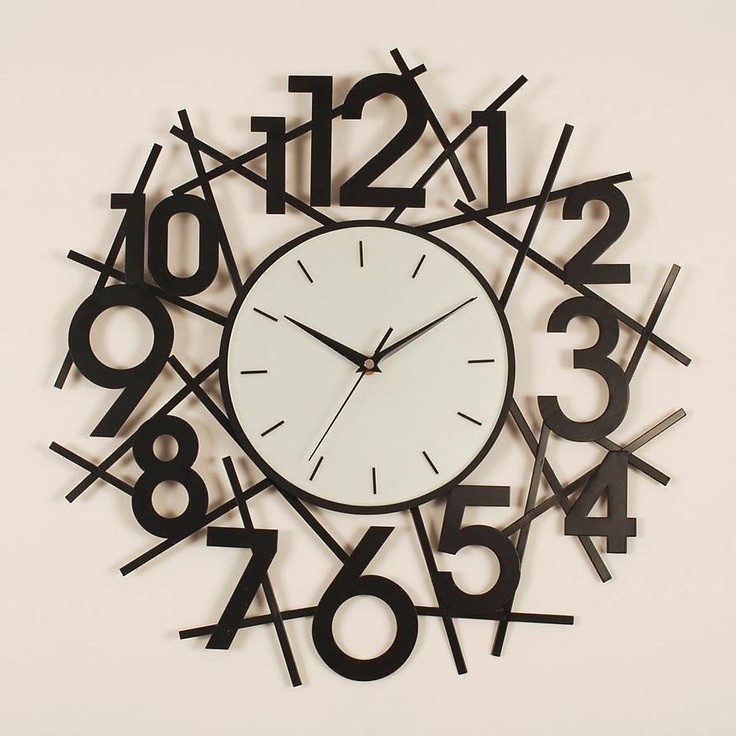This image showcases a uniquely designed clock mounted on a flat, white wall. The clock features a minimalist, circular face with a pristine white background. Instead of traditional numerals, the face is marked with simple lines to denote the hours. The time is indicated by three distinct hands: an hour hand, a minute hand, and a second hand. Adding to its distinctive appearance, the clock incorporates a set of numerals placed outside the circular face. These numerals vary in size, larger at certain points and smaller at others, and are set within a sleek, metallic framework that outlines the face. The overall design combines functionality with artistic elegance, making it a striking focal point on the plain white wall.